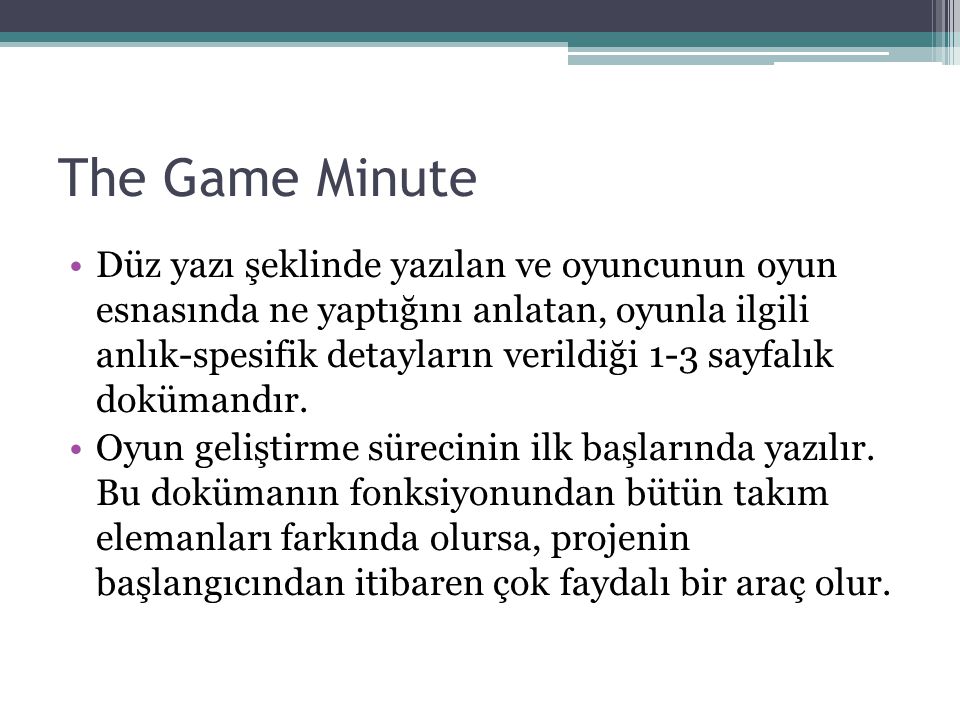The image features a prominent banner at the top transitioning from dark green to light green with subtle white streaks towards the right edge. Beneath this banner, the background is completely white. At the top of this section, the title "The Game Minute" is displayed in a light black, slightly faded text. Below the title, there are two paragraphs of text, each consisting of four lines and marked by pink bullet points. The text within these bullet points is in a foreign language and both paragraphs conclude with a period.